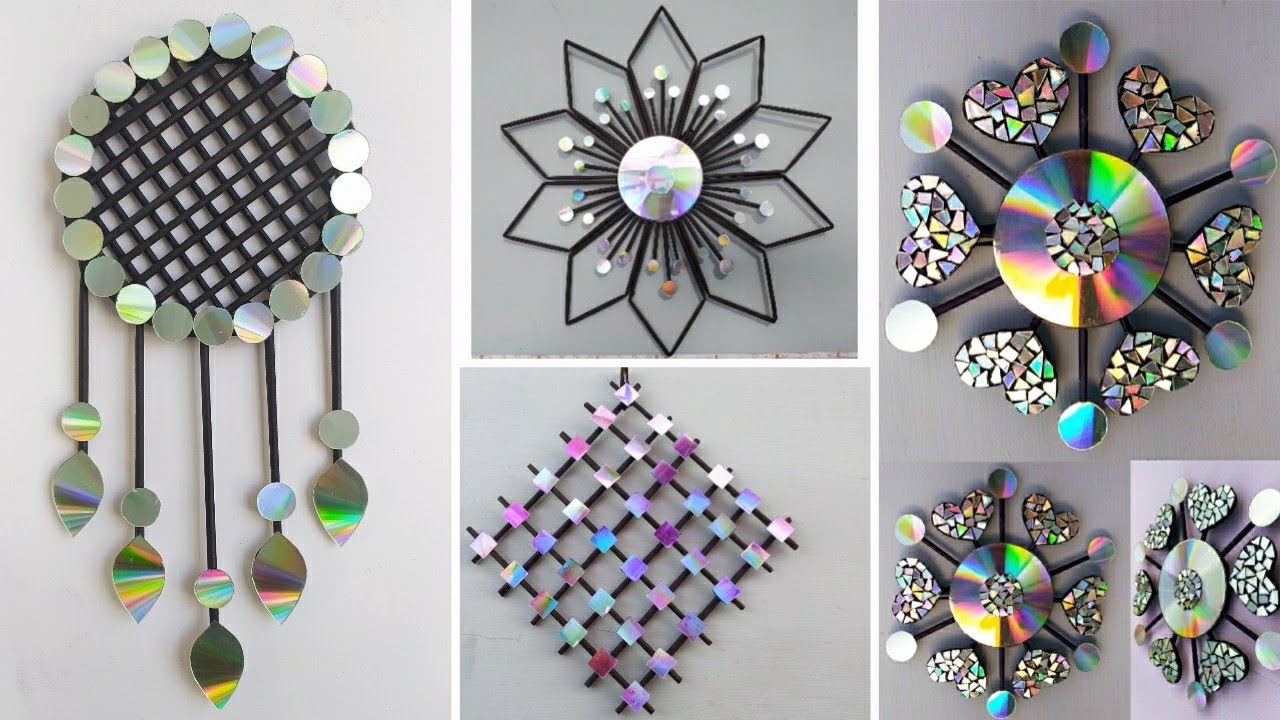This image is a detailed collage of six distinct pieces of wall art, all set against a grayish-blue background and arranged in various sizes to form a single large, cohesive photograph. The largest piece, on the left, resembles a dreamcatcher, featuring a central black netted circle bordered by shiny, mirrored circles and reflective black strings with dangling elements at the end. To its immediate right is a flower-like design that employs the same reflective, rainbow-hued materials as the dreamcatcher.

Below the flower is a grid-like sculpture consisting of reflective, purplish squares arranged in a woven pattern. Adjacent to this sculpture on the right is a circular piece resembling a clock, made from the same black and mirrored materials. This design radiates black lines and is adorned with small hearts and reflective circles, creating a clock-like appearance.

To the bottom right of the "clock" are two similar circular pieces. The left one appears as if it might be constructed from an old CD, incorporating reflective, mirror-like elements shaped into various forms such as circles and hearts. The rightmost piece displays a centralized circle with six hearts and six lollipop-shaped extensions, all employing the consistent mirrored and reflective materials seen throughout the collage.

This cohesive arrangement of reflective wall decor pieces highlights intricate designs and materials, creating a unified aesthetic theme focused on shiny, reflective, and rainbow-iridescent elements.